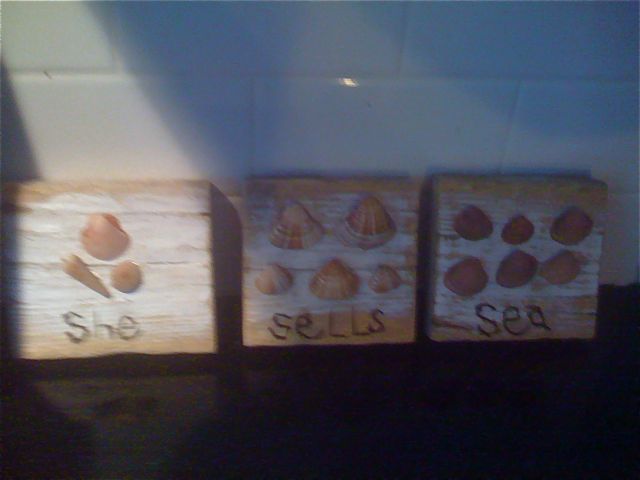The photograph, slightly out of focus, captures a scene featuring a dark, almost black countertop set against a shiny white subway tile backsplash. Three decorative displays, likely mounted on wooden boards with tan tops and bottoms, rest on the countertop, each adorned with seashells of various shapes and sizes—flat, oval, pointed, and triangular—reminiscent of those found on the beach. These displays form a visual play on the tongue twister "She sells sea shells," with each board featuring white paint and black handwritten text. The first board, illuminated by a light that casts a reflection on the countertop, reads "SHE" and is decorated with three shells. The second board, labeled "CELLS," showcases five shells. The final board contains the word "SEA" and is adorned with six shells. The overall effect evokes a collection of beach memories meticulously arranged on tiles for decorative purposes.